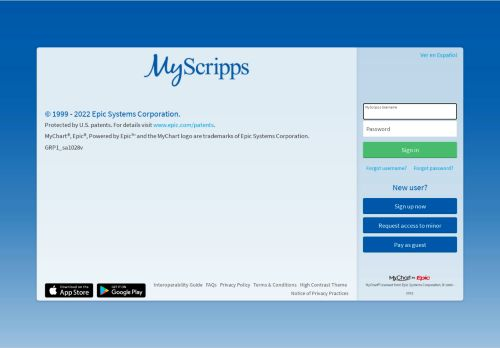The webpage features a gradient background that transitions from bright blue at the top to light blue towards the bottom. Overlaid on this background is a smaller rectangular section, which occupies the far right quarter of the page and is filled with a medium blue color. 

Within this smaller section, there are two input fields at the top: one for entering a username and the other for a password. Below these fields is a prominent green "Sign In" button. Just beneath the sign-in button, a line of text in blue ink reads "New User?".

Below this section, there are three dark blue buttons with various functionalities: "Sign Up Now," "Request Access," and an ambiguously worded button that likely reads "Pay as Guest" or "Try as Guest."

At the top left of the page, there is a lighter gray box containing the text "MyScripps." The word "My" is written in cursive, while "Scripps" (spelled S-C-R-I-P-P-S) is in standard text. Beneath this, it states "1999 to 2022 Epic Systems Corporation." Below this text is additional smaller text that is too tiny to read.